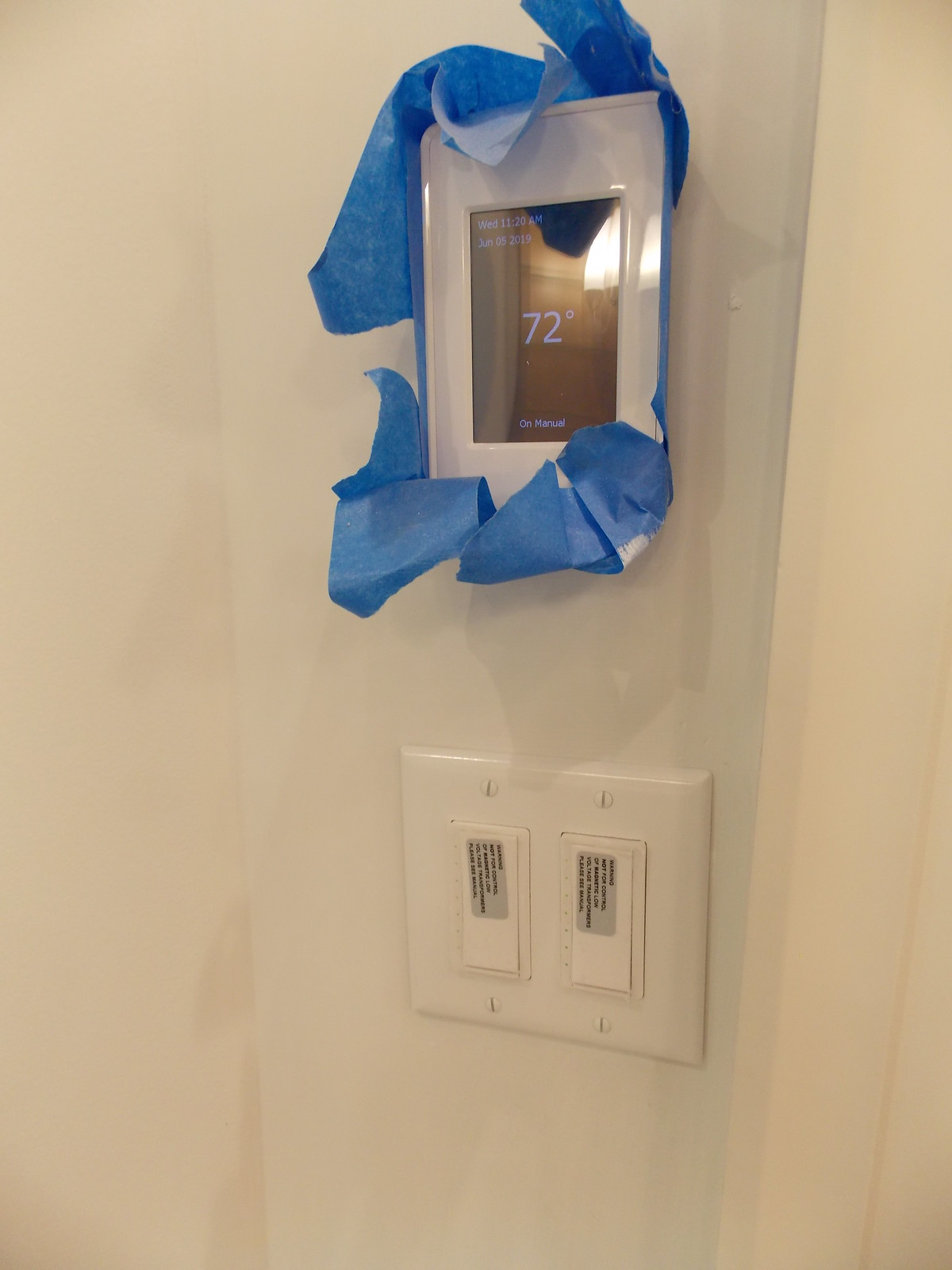In the image, there is a newly installed thermostat situated in a recently constructed area. Blue tape surrounds the thermostat, likely protecting the adjacent wall during the remaining construction work. The thermostat, featuring an LED screen encased in a white frame, displays a temperature setting of 72 degrees. Additional information on the screen includes the date and time: "Wednesday 11:20 a.m., June 5th, 2019," and an operation mode labeled as "Manual." Below the thermostat, there are two toggle-style light switches, each with small stickers that have not yet been removed, indicating their new installation status. The blue tape around the thermostat and the stickers on the switches suggest that final touches and adjustments are still pending in this construction project.